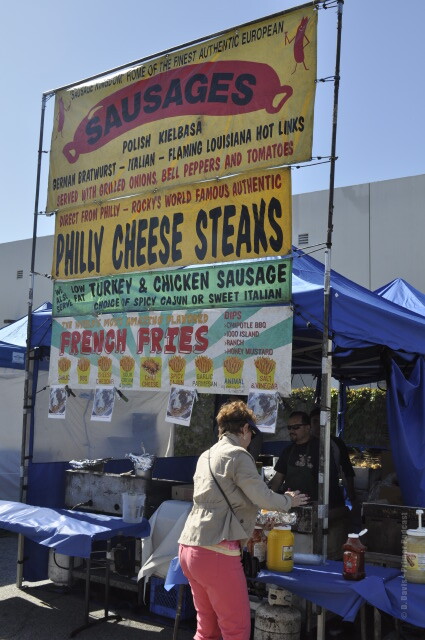This photograph captures a bustling outdoor food venue, particularly focusing on a vibrant blue tent with a rich variety of offerings prominently displayed on its signage. The top of the booth’s sign showcases a diverse selection of sausages, including Polish sausages, German bratwurst, and Italian varieties, alongside Spicy and Cajun as well as sweet Italian options, with flaming Louisiana hot links served with broiled onions, bell peppers, and tomatoes. Just below, the sign boasts Rocky's world-famous authentic Philly cheesesteaks. Further down, the sign highlights healthier choices such as low-fat turkey and chicken sausages. The mention of "world famous french fries" is prominently illustrated with images of numerous batches of fries below this description.

In the scene, a woman appears to be preparing to add mustard to her food item, though the item itself is not visible in the photograph. Surrounding her are jars of condiments including ketchup. Additionally, a man wearing sunglasses stands inside the tent, seemingly serving food to customers. The details and atmosphere suggest a lively and appealing food venue offering a delightful array of comfort foods.